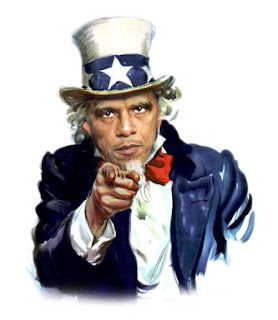The image features a depiction of Uncle Sam with distinct characteristics. He wears a traditional white hat adorned with a blue band and white stars. His attire includes a blue jacket that transitions in shade from dark navy on the left to a lighter blue on the right, complemented by a white shirt and a partially visible red bow tie. Uncle Sam's white hair and beard frame his face, which has notably darker skin and a resemblance to Barack Obama. His face is marked by piercing eyes and heavy eyebrows. Notably, there is an unexpected splash of green on his shirt, intertwined with blue lines. The hat has shadows that give parts of it a gray appearance. Uncle Sam's right hand extends forward with an accusatory finger pointing directly at the viewer, with a tiny dot of red from the bow tie visible near his hand. The overall image is detailed and encapsulates both traditional and unique elements of Uncle Sam's iconic look.